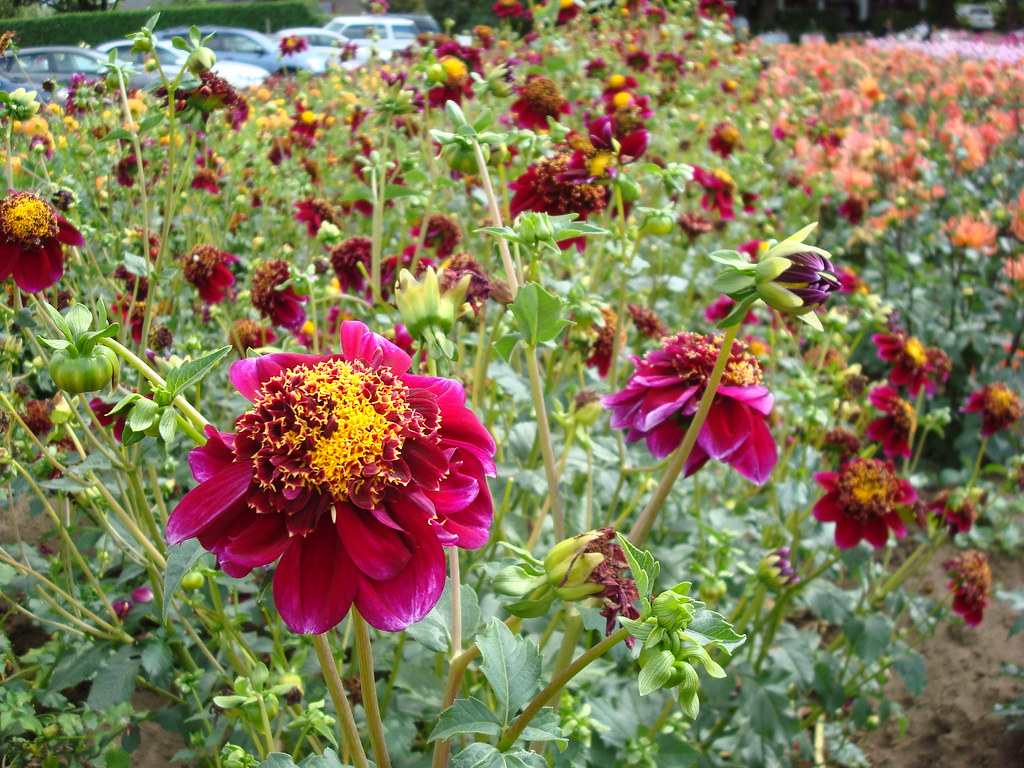This landscape image prominently features a close-up of a vibrant wildflower garden. In the foreground, the focus is on a lush, large pink flower with magenta petals, accented by a bushy middle of yellow and maroon stamens. To the right, a smaller flower of the same variety appears, slightly less magnified. Scattered throughout the scene are numerous maroon-colored flowers with vivid yellow pollen at their centers. The background, which is more blurred, showcases clusters of pink flowers. Off to the right side, the blurriness makes it difficult to distinguish some flowers, which appear to be yellowish or orangish. The upper left corner of the image reveals a line of five parked cars next to a long green bush, suggesting that this picturesque flower patch is located near a public area or parking lot. Additionally, a small patch of dirt is visible in the lower right corner, adding a touch of natural texture to the scene.